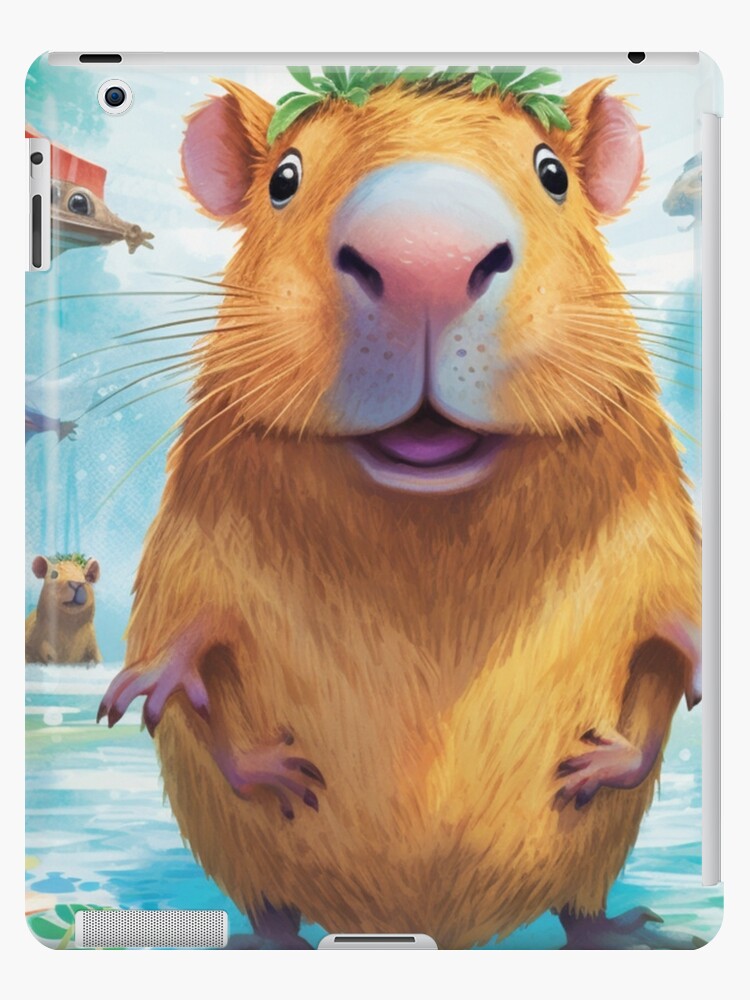This image showcases a very cute, slightly deformed cartoon hamster that would be perfect for a children's book about animals. The hamster, tan in color with black and white eyes that give it a happy and perky look, takes up most of the space in this square image. It's depicted on the back of an iPad case, creating a charming design. This hamster has some unique features: two arms emanating from the same joint on its left side, a pink nose with white highlights, tiny yellow whiskers, and a slightly open mouth revealing a pink tongue. The inside of its ears is pink and it wears a small crown of green leaves on its head. The backdrop is a blue water scene. To the left side of the hamster is another brown, partially submerged creature, possibly another hamster or guinea pig. Additionally, in the upper left-hand corner, there is a small faint image of an amphibious animal, potentially a snake or lizard, wearing what appears to be an orange bottle cap.